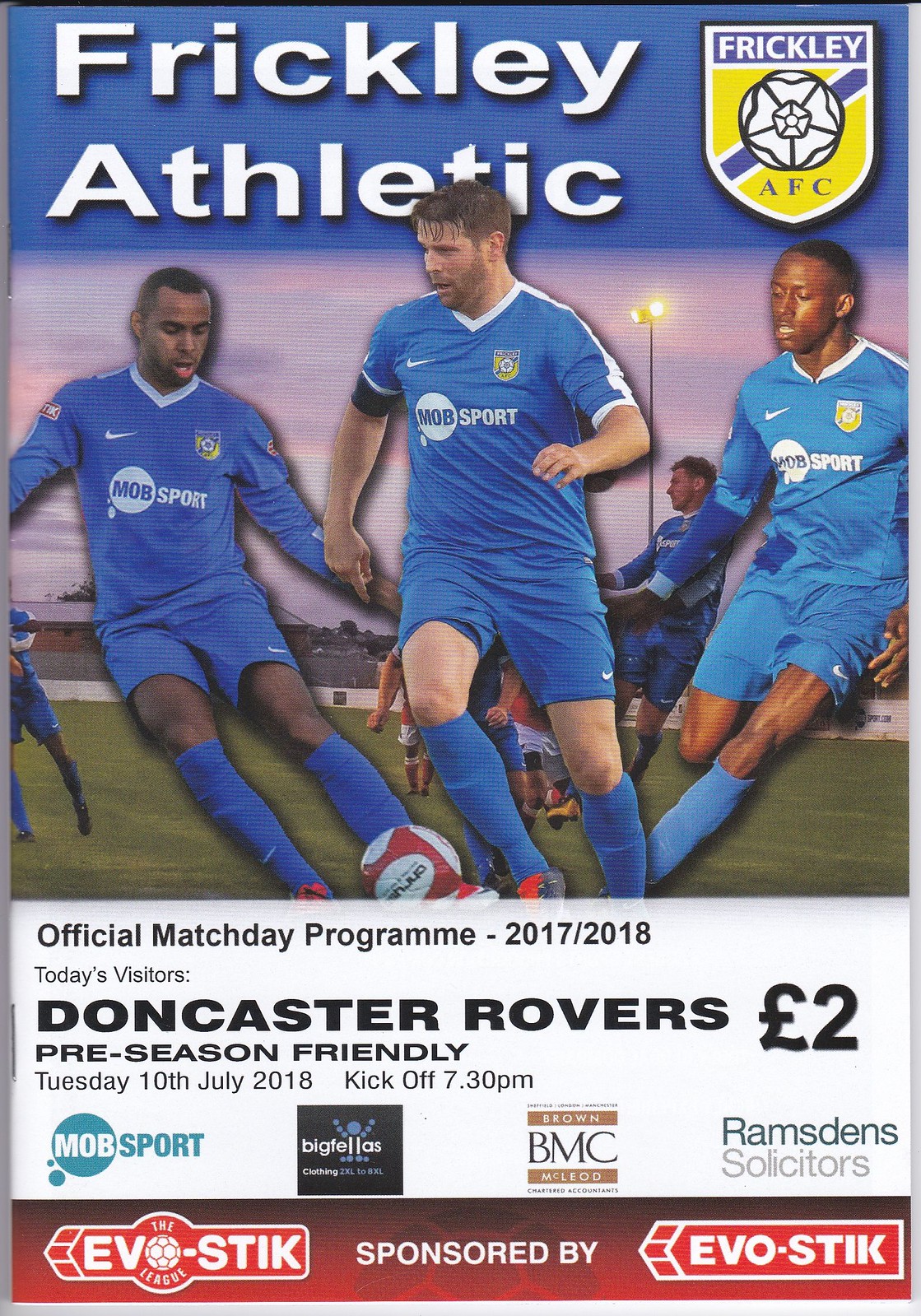This detailed image depicts the front cover of an official match day program for the 2017-2018 season of Frickley Athletic F.C., a soccer team. At the top of the cover, a blue stripe features the white text "Frickley Athletic." In the right corner, there's a shield-shaped club logo with the word "Frickley" in white at the top, a white and black soccer ball in the center, a blue diagonal stripe, and a yellow background. Below the logo, it reads "AFC."

The center of the cover showcases an action shot of three players superimposed on an image of a soccer field. The players, dressed in blue uniforms with the sponsor name "Mobsport," include two African American men and one Caucasian man. Each player is equipped with blue shin guards and features additional branding such as a white Nike logo and a white circle on their jerseys.

The bottom third of the cover is a white rectangular area with essential event details: "Official Match Day Program 2017-2018," "Today's Visitors, Doncaster Rovers," "£2, Preseason Friendly," "Tuesday 10th, July 2018, kickoff 7.30pm." Below these details are the logos of various sponsors, including Mobsport, Big Fellas, BMC (Brown McLeod), and Ramsden Solicitors. The program is sponsored by Evo-Stik, featuring a red and white logo with a soccer ball replacing the 'O' in "Evo".